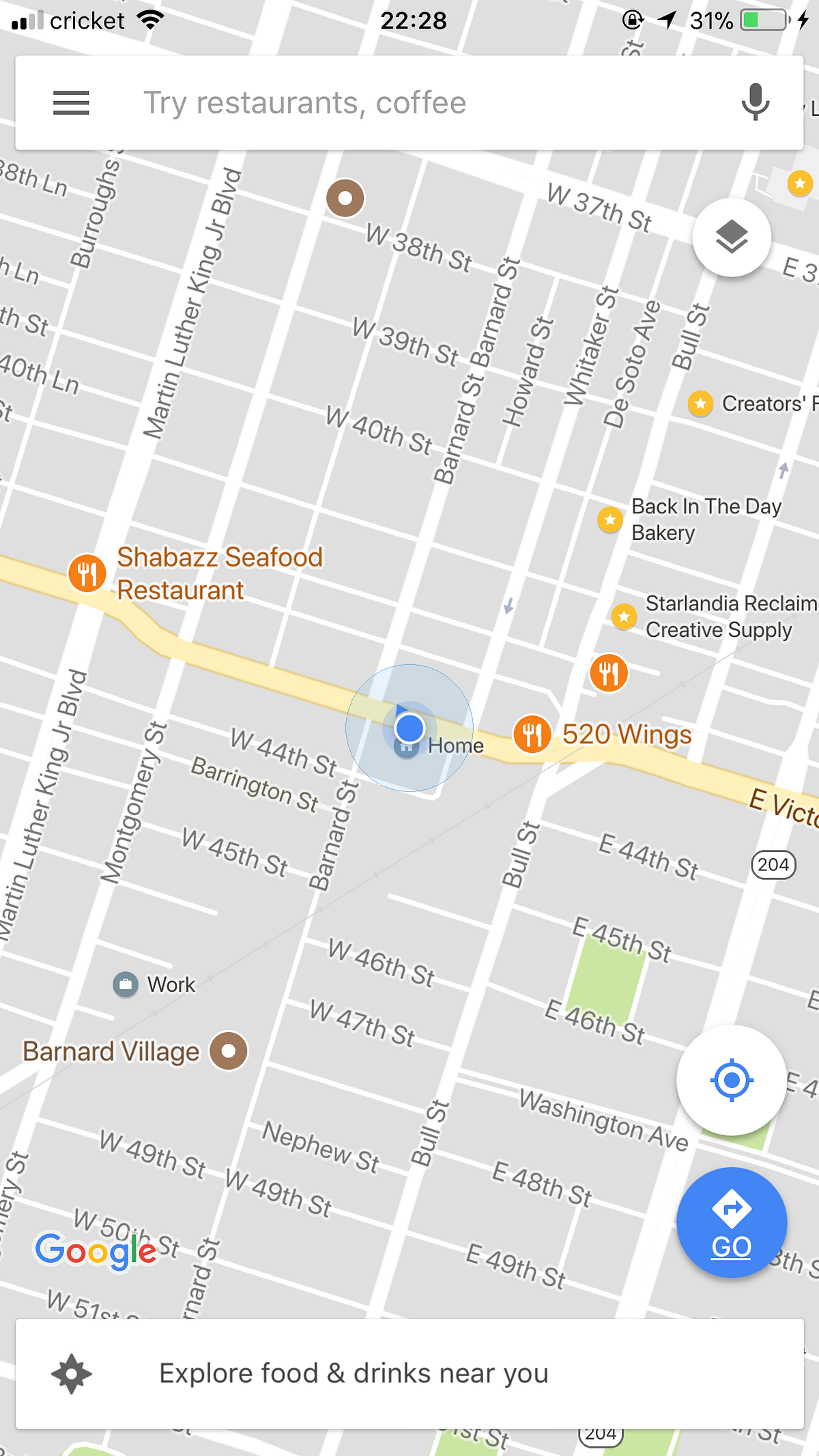An image captured on a smartphone screen displaying a navigational map interface. At the top of the screen, the search bar contains the text "Try restaurants, coffee." The map shows a network of white roads, with a prominent yellow road running through the center. Near the label "Home," a radar-like blue circle indicates the user's current location.

Several notable points of interest are marked, including Shabazz Seafood Restaurant, 520 Wings, and Barnard Village. Street names such as East 49th Street, East 48th Street, East 45th Street, East 46th Street, and up to West 37th Street are clearly visible. A significant thoroughfare, Martin Luther King Jr. Boulevard, is also highlighted.

Restaurants are denoted with icons featuring a fork and knife within reddish-orange circles. Toward the lower section of the screen, there is a blue "Go" button with a turning arrow symbol, indicating a navigation option. At the bottom, a white bar offers the action "Explore food and drinks near you."